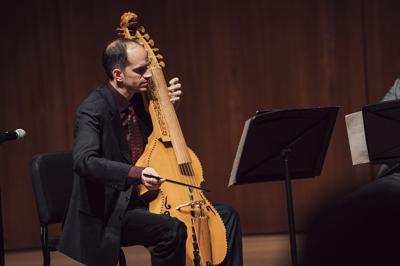The image captures a man seated on a black chair, meticulously playing a cello, this large stringed instrument held upright with his left hand while he skillfully maneuvers a bow across its strings with his right hand. He is intently focused on sheet music positioned on a black stand directly in front of him. Dressed in a nicely tailored black suit with a red undershirt and tie, the man sits on a stage, exuding an air of formality and dedication. He is bald on top with Caucasian features, and a few elements like a microphone on the left and some brown drapes in the background partially visible, hint at an orchestral setting. The scene is bathed in a palette of black, beige, burgundy, and brown, complementing the polished wood of the cello and creating a classical, refined atmosphere. Though other performers seem to be present, they are not distinctly visible in the image.